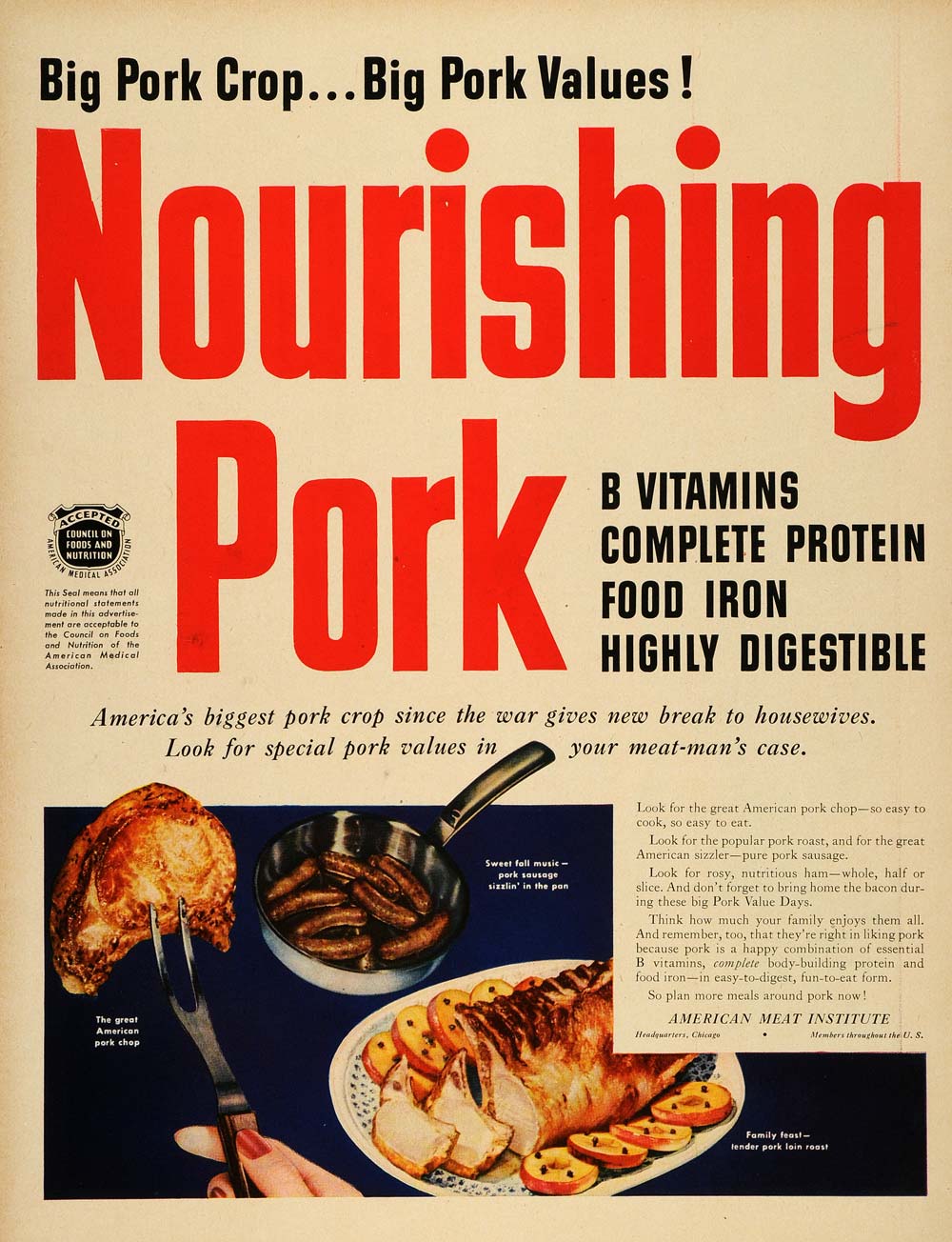The image appears to be an old advertisement page from a magazine or a cookbook, featuring a light pink or beige background. At the top, large black letters proclaim "Big Pork Crop, Big Pork Values," followed by bold red text stating "Nourishing Pork." Beneath this, benefits of pork are listed: "B Vitamins, Complete Protein, Food Iron, Highly Digestible." The advertisement includes a smaller headline reading, "America's Biggest Pork Crop Since the War Gives New Break to Housewives," followed by, "Look for Special Pork Values in Your Meat Man's Case." The bottom section showcases colorful drawings of various pork dishes against a dark blue background, including a white plate filled with pork, a metal pan with browned pork sausages, and what appears to be a pork tenderloin with pineapple. To the left, a hand holding a fork with meat is visible. An article in black text is positioned on the right side of the images.